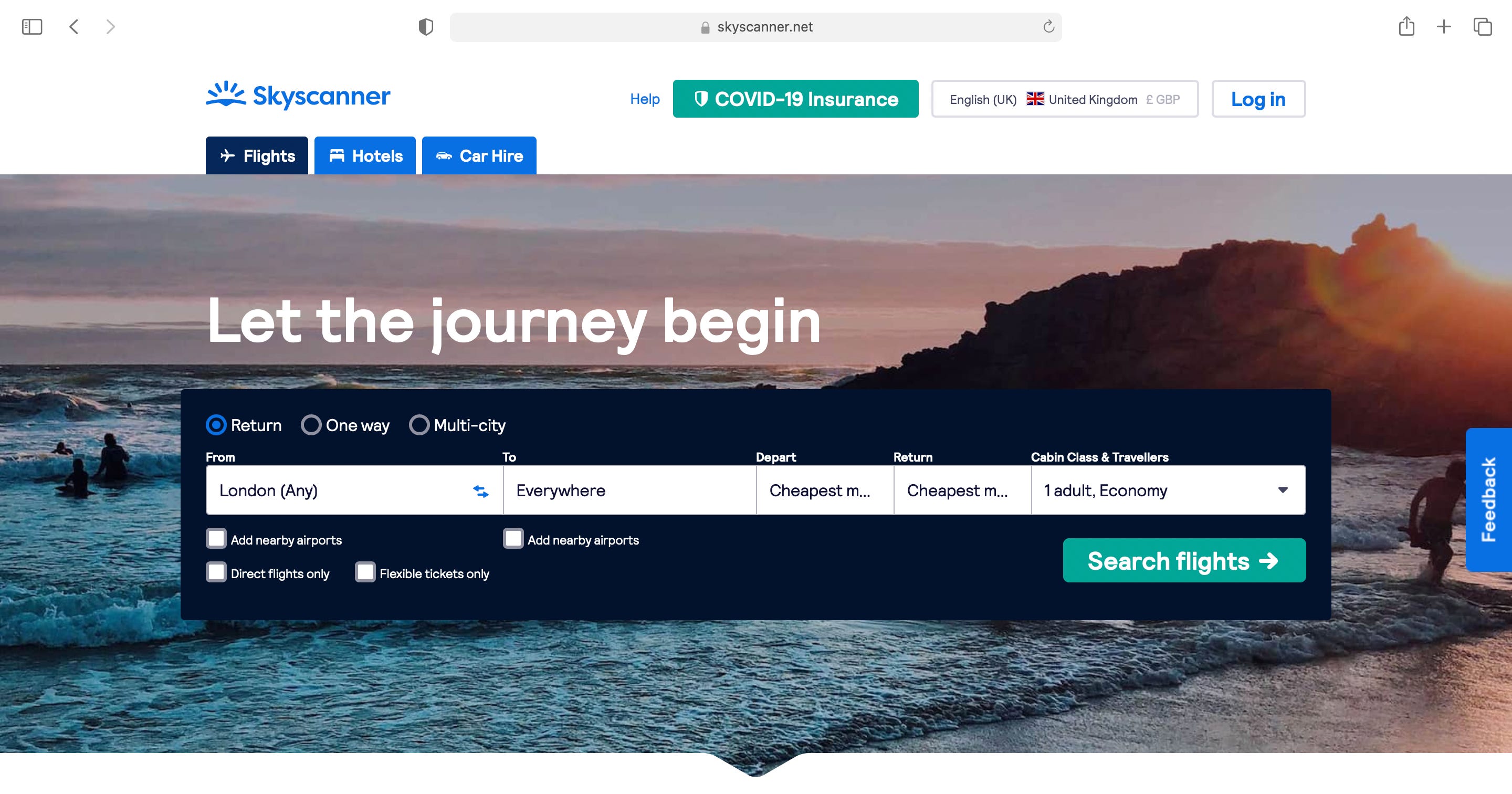The image is a screenshot of a Skyscanner flight search webpage. The interface is presented horizontally, and the overall image is a bit wider than a standard landscape orientation. The background is predominantly white.

At the top of the page, there is a search bar that reads "skyscanner.net". On the left side, the Skyscanner logo is visible, featuring an icon of a sun rising over a blue horizon. Adjacent to this, in blue text, it says "Help". There's also a green button labeled "COVID-19 insurance" in white font, accompanied by a shield icon. Further to the right, there is a white button labeled "English (UK)" with an icon of the UK flag. It also displays "United Kingdom" and "GBP". Next to this button is a blue rectangular button that says "Log in".

Beneath this top bar, there are three tabs on the left: a navy blue one labeled "Flights", and two royal blue ones labeled "Hotels" and "Car Hire", each with their corresponding icons.

Below these tabs, there is a wide image of a beach at sunset. The image depicts waves rolling in and people playing near some rocks in the background. Overlaid on the image in white text are the words "Let the journey begin".

At the bottom of this section, a navy blue horizontal bar presents search options. The options visible include "Return", which is currently selected, alongside "One-way" and "Multi-city". The search inputs indicate "From: London" and "To: Everywhere", with dropdown suggestions showing "Depart: Cheapest month" and "Return: Cheapest month".